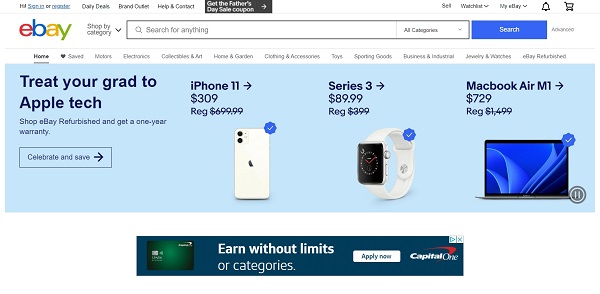The image depicts a webpage from eBay, capturing various elements of its interface. In the upper left-hand corner, the iconic eBay logo is prominently displayed, featuring a red 'e', blue 'B', gold 'a', and green 'y'. 

At the top of the page, there are navigational categories that include options like "Daily Deals," "Brand Outlet," and "Help & Contact." Nearby is a black box highlighting a Father's Day coupon offer. The top menu also includes links to a watch list, "My eBay," a shopping cart alert, and a "Sell" button.

Below the top menu is a gray-outlined search bar allowing users to search across all categories. Adjacent to the search bar is a blue "Search" button and an "Advanced" search option.

In the center of the webpage is a light blue rectangular box detailing a promotional event, encouraging users to "Treat your grad to Apple Tech." The promotion features a button labeled "Celebrate and Save" and mentions the benefits of shopping eBay Refurbished, including a one-year warranty. Featured products include an iPhone 11 priced at $309 (down from $699), an Apple Watch Series 3 at $89.99 (down from $399), and a MacBook Air M1 at $729 (down from $1499). Accompanying each product listing is an image of the respective item.

Beneath this promotional box is another section promoting a Capital One offer. This dark gray box discusses earning benefits without limits or categories and includes an image of a green Capital One card on the left-hand side. An "Apply Now" button is prominently displayed.